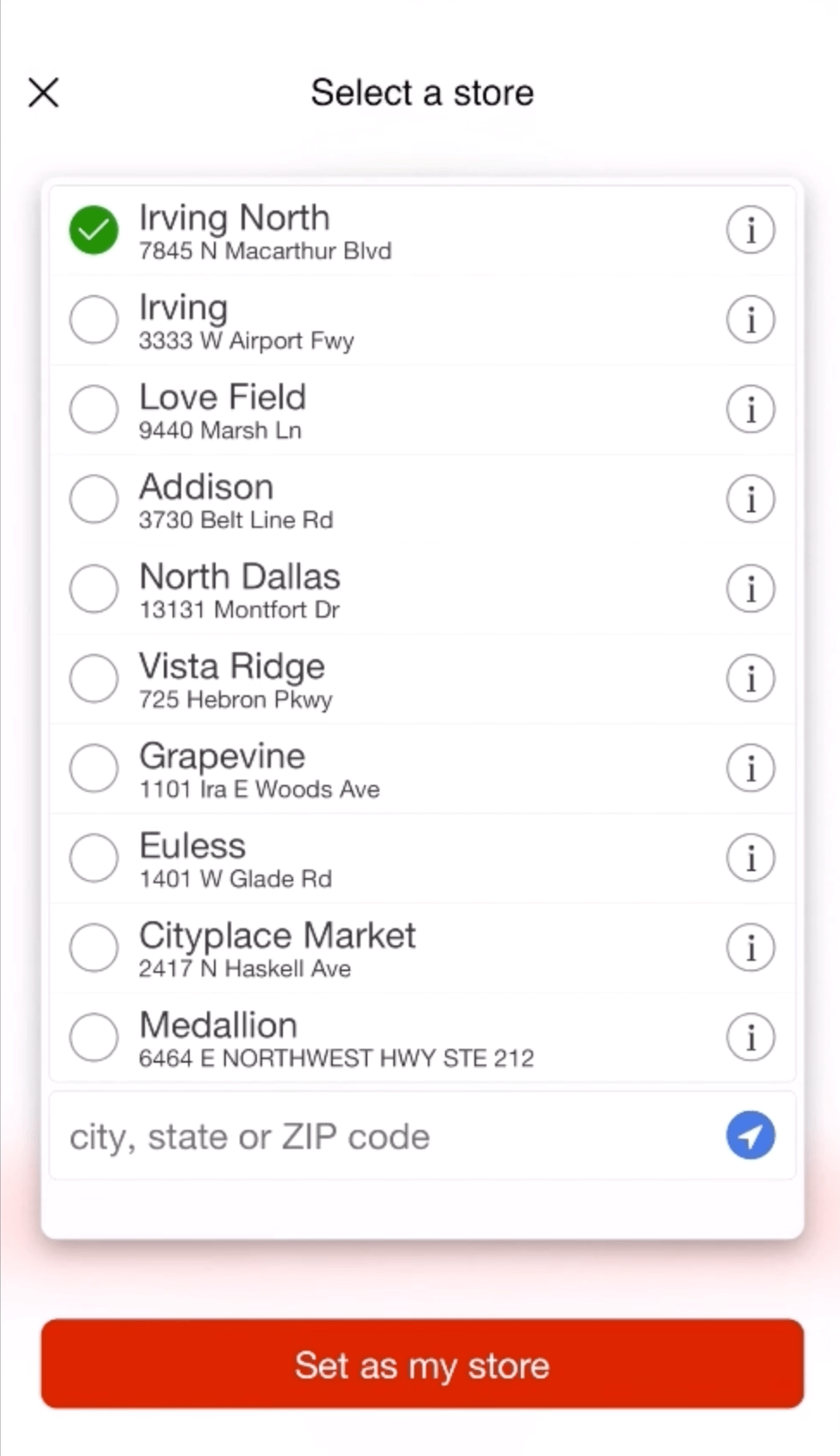The image depicts a mobile application interface for a store locator feature. The interface appears to have multiple tabs, with the current tab focused on store locations. On the right side of the tab label, there is an 'X' button, likely used to close the tab.

Prominently displayed in the central part of the screen is a list of store locations. Each location entry includes the name of the store and its detailed address below it. The listed locations are: Irving North, Irving, Love Field, Addison, North Dallas, Vista Ridge, Grapevine, Euless, City Place, Market, and Medallion.

Adjacent to each store name is a circular checkbox, enabling users to select a store. The first store, Irving North, is currently selected, as indicated by a checkmark within the circle.

At the top of the list, there is a text field labeled "Search for city, state, or zip code," allowing users to input their desired search criteria to find a relevant store. Below this search field, there is a large rectangular button labeled "Set as My Store," providing an option to designate a preferred store.

To the left of the store list, various icons that resemble eyes are visible, possibly representing settings or views related to the store selection process.